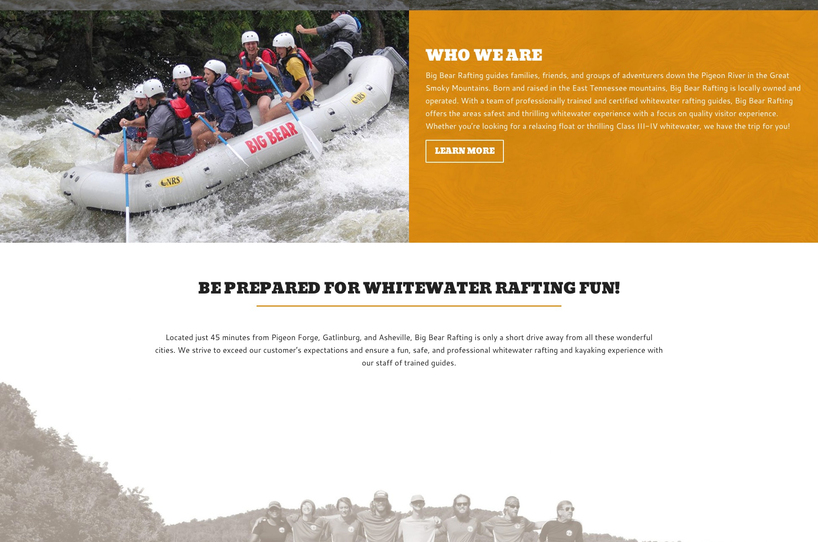Big Bear Rafting Advertisement

Discover the thrill and adventure of Big Bear Rafting as they take families, friends, and groups down the scenic Pigeon River in the beautiful Great Smoky Mountains. Proudly born and raised in the East Tennessee Mountains, Big Bear Rafting is a locally owned and operated company with professionally trained and certified white-water rafting guides.

Experience the area's safest and most exhilarating water adventure, with a strong emphasis on quality and safety. Whether you’re seeking a relaxing float or an adrenaline-pumping journey through Class III to IV rapids, Big Bear Rafting has the perfect trip tailored for you. 

In the image, adventurous participants can be seen enjoying the thrill of white-water rafting in sturdy inflatable rafts, equipped with durable plastic oars. Each rafter wears a white helmet and a life jacket to ensure maximum safety and an unforgettable experience. 

At the bottom of the advertisement, further information is provided under the header "Prepare for White Water Rafting Fun," guiding potential adventurers on what to expect and how to get started. To learn more about the exciting trips and excellent customer service, simply click "Learn More" on the left of the advertisement.